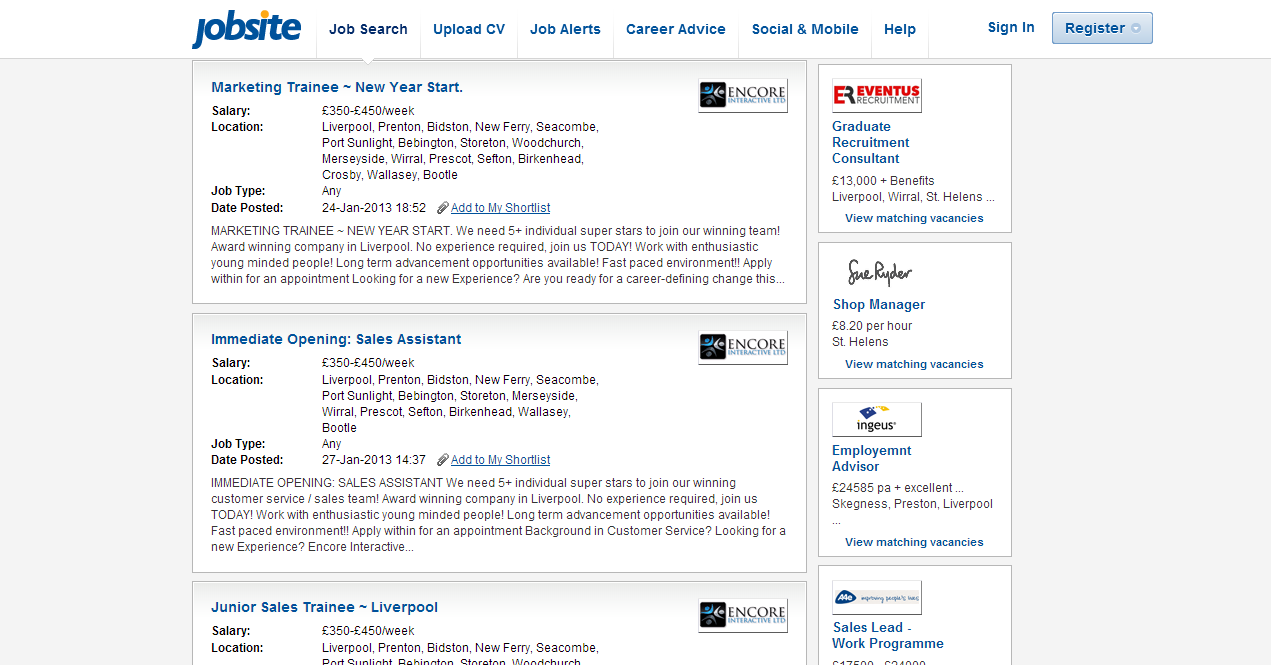In the image, there is a user interface for a job-search platform. At the top-left corner, there is the title "Job Site." Moving right from the title, a navigation bar includes links for "Job Search," "Upload CV," "Job Alerts," "Career Advice," "Social and Mobile," "Help," and "Sign In." At the far right, there is a prominent light blue button labeled "Register." All of these links and the button are styled in light blue.

Below the navigation bar, the first job listing is for "Marketing Training, New Year Start," offering salaries between £350 to £450 per week. The location includes several areas: Liverpool, Prenton, Byston, New Ferry, Seacombe, Port Sunlight, Bevington, Stornton, Woodchurch, Merseyside, Wirral, Prescott, Sefton, Birkenhead, Crosby, Wallasey, and Bootle. The job type is labeled "Any" and it was posted on 24th January 2013 at 18:52. There is an option to "Add to my shortlist." The listing mentions the need for five or more "individual superstars" to join their winning team.

The next listing is for an "Intermediate Opening Sales Assistant," with a salary range of £350 to £450 per week. The job locations include Liverpool, Prenton, Byston, New Ferry, Seacombe, Port Sunlight, Bevington, and Shorton. This job type is also labeled as "Any," and it was posted on 27th January 2013.